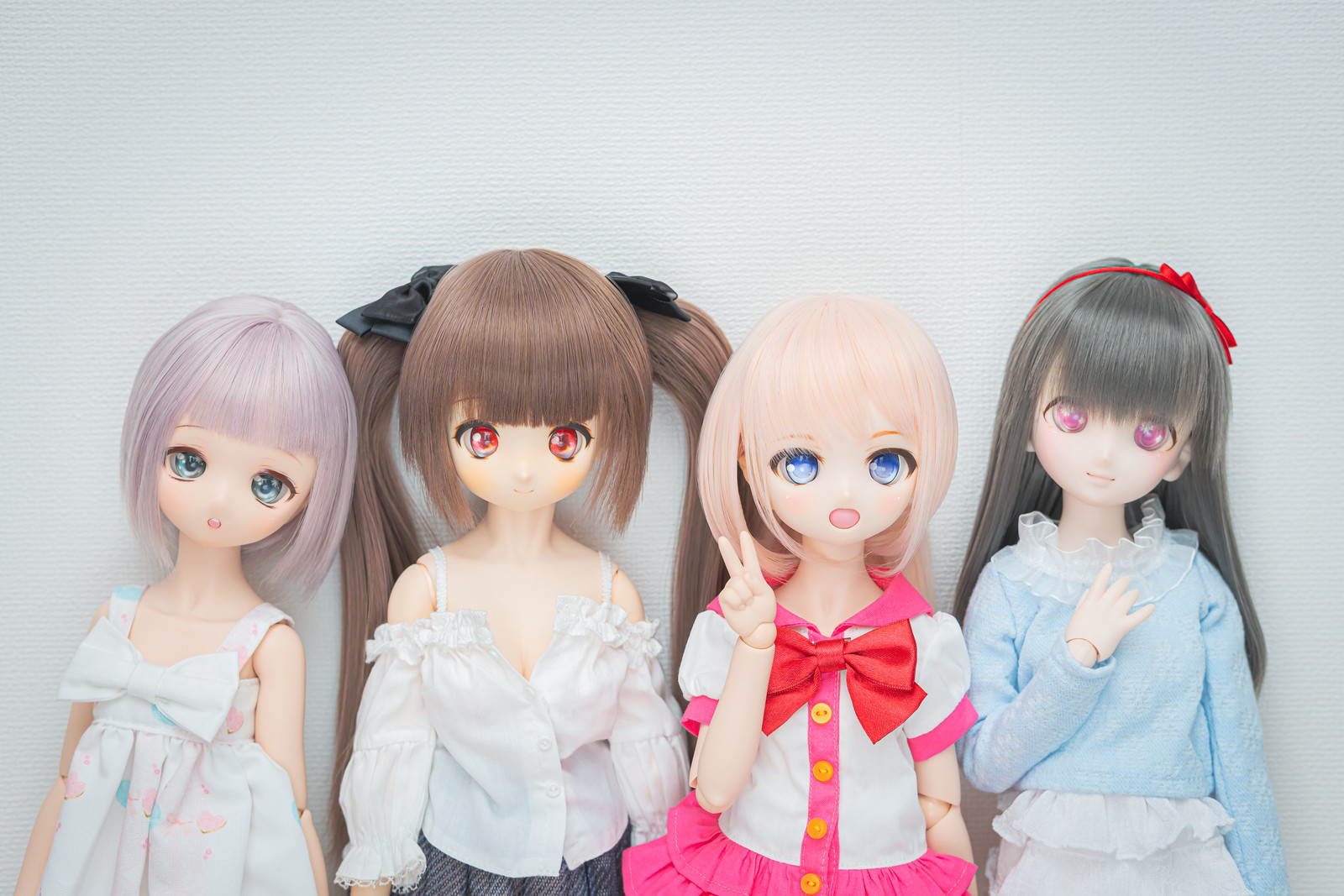The image showcases four anime-styled dolls, visible from the waist up, set against a white background. These dolls have large, exaggerated eyes typical of anime characters, with each sporting unique hair colors and styles. Starting from the left, the first doll has short, light purple hair and big blue eyes, dressed in a sleeveless pastel pink and blue dress adorned with a large bow at the front. The second doll features long brown ponytails tied with black bows and has reddish-brown eyes. She wears a white blouse with sleeves cascading off her shoulders, hinting at a skirt beneath. The third doll has short, light blonde hair and bright blue eyes, dressed in a white dress accented with pink ruffles and a big red bow, complete with yellow buttons. The fourth doll has long, straight grayish-brown hair, decorated with a red ribbon headband. Her large eyes are a purplish-pink hue, and she wears a blue sweater with a ruffled collar over a skirt with visible ruffled layers. The entire image is brightly lit, emphasizing the light-colored clothing and detailed designs of the dolls.